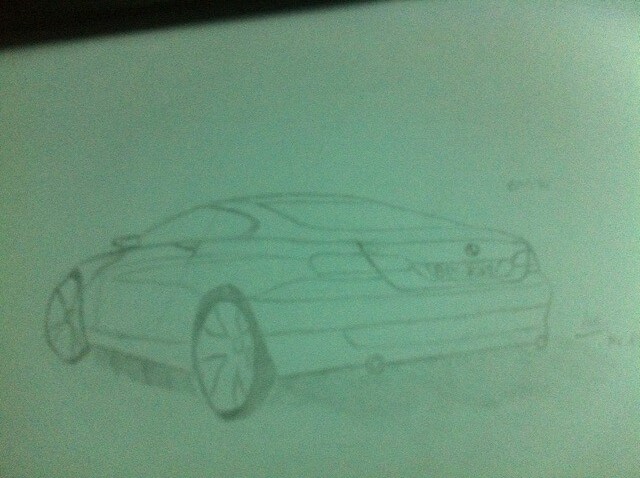This is an image of a photograph depicting a detailed pencil drawing on greenish-yellow tinted paper, possibly due to poor lighting. The photograph captures a back and side view of a sleek sports car, likely a Mercedes-Benz based on the indistinct logo and high-level detail, though there is some speculation it could be a BMW or Lexus. The car is a two-door coupe, prominently showing the driver's side with a visible side mirror and a door handle. The trunk and license plate are distinct, although the characters on the plate are unreadable. The car appears to be in motion, suggested by shaded areas underneath the vehicle and slight indications of smoke. The realistic rendering includes black tires with silver or metallic rims and well-defined shading, enhancing the lifelike quality of the drawing. The top left corner of the image transitions into a curved black area, possibly indicating the photo was taken while the paper was held up, adding a dynamic element to the scene. Overall, the artwork impressively captures the sporty essence of the car, making it the focal point against the subdued backdrop.